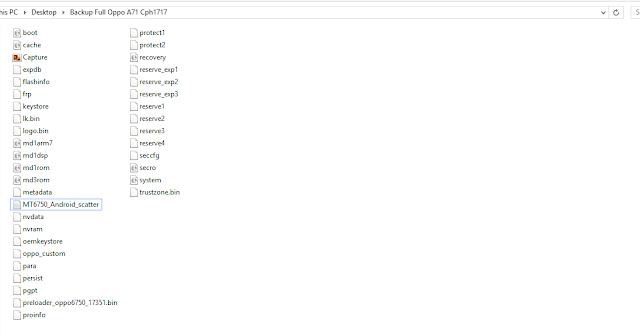The image displays a computer interface, specifically a file explorer window. At the top of the window, a path is visible, indicating the location: "This PC > Desktop > Backup for OPO 871 CPH 1717". Below this path, the window is divided into two columns.

Each line in these columns presents an icon on the left side and an input box on the right. The icons appear to represent different file types or system resources. The list on the left side from top to bottom includes the following file names:

1. boot
2. cache
3. capture
4. AXP
5. DB
6. flash info
7. FRP
8. key store
9. LKBIM
10. logo.bin
11. MD1ARM7
12. MD1DSP
13. MD1ROM
14. MD3ROM
15. metadata
16. MT6750
17. NV_Android_scatter
18. NV_data
19. NV_TAM
20. OEM
21. keystone
22. oppo__custom

Each file appears to be associated with specific functions or components necessary for system operations or device backups, likely related to an Oppo smartphone model. The organized presentation suggests it may be used for advanced tasks such as firmware updates or custom ROM installations.